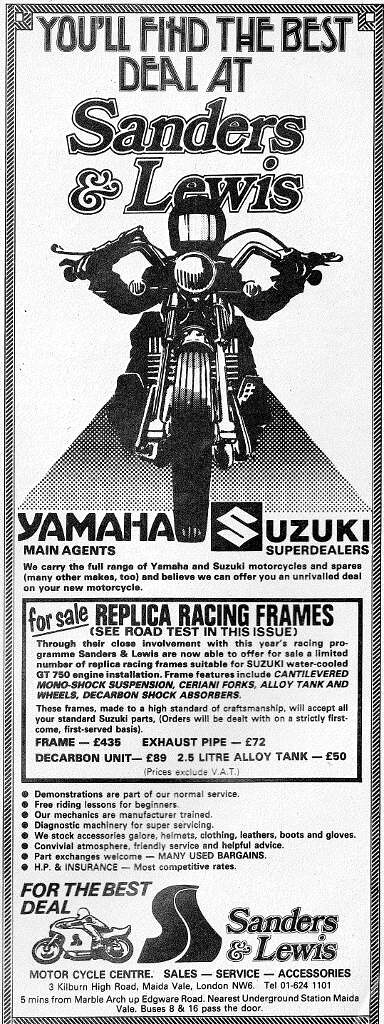This is a detailed black-and-white advertisement for Sanders and Lewis, renowned dealers for Yamaha and Suzuki motorcycles. The ad features a prominent drawing of a motorcyclist wearing a helmet, riding towards the viewer, with a checkered triangle in the background. The headline boldly declares, "You'll find the best deal at Sanders and Lewis." Below this illustration, it emphasizes their role as Yamaha main agents and Suzuki super dealers. A side panel highlights a special offer: "For sale: replica racing frames - see road test in this issue," indicating the ad's placement in a motorcycle magazine. The lower section of the ad details their extensive services, including demonstrations, free riding lessons for beginners, and a team of manufacturer-trained mechanics. The dealership's London address, telephone number, and directions are provided at the bottom, alongside an additional drawing of a motorcycle, reinforcing the ad's focus on high-quality motorcycle deals and services.